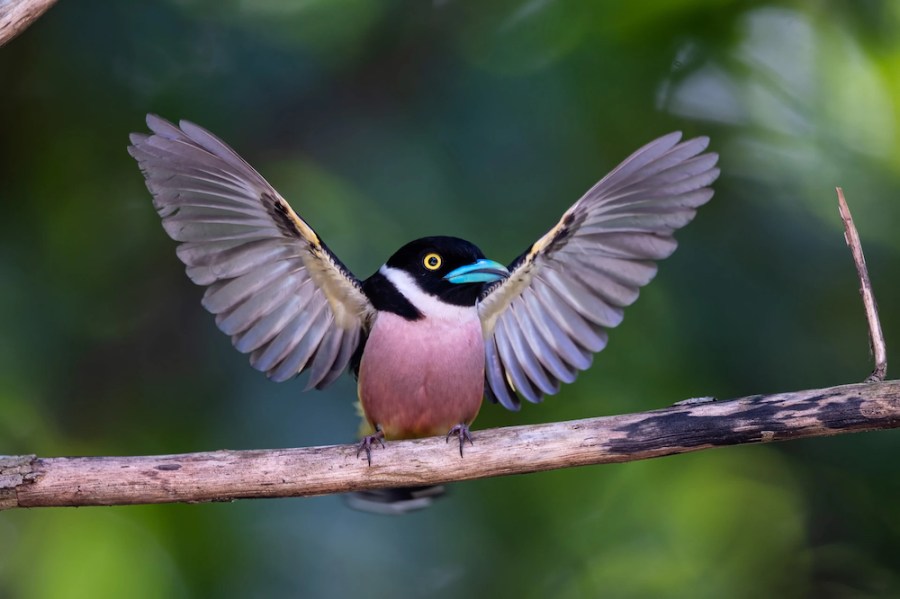The horizontal rectangular photograph captures a vibrant and colorful bird perched on a bare wooden branch, with its wings outstretched as if it just landed or is about to take off. The bird's distinct features include a black head, a bright turquoise beak, and striking yellow irises encircling its black pupils. A white collar encircles its neck, with the black coloring continuing onto its back. Its chest displays a vivid rosy red hue, while the wings showcase an intricate pattern of gray and grayish-blue feathers, with brown near the attachment points. There's also a glimpse of pale purple and yellow on the wing's underside. The bird's dark gray feet tightly grip the branch. In the background, a green blur suggests a lush, outdoor setting, possibly in spring or summer. The branch, devoid of bark, has an additional offshoot with a few leaves, complementing the natural beauty of the scene.